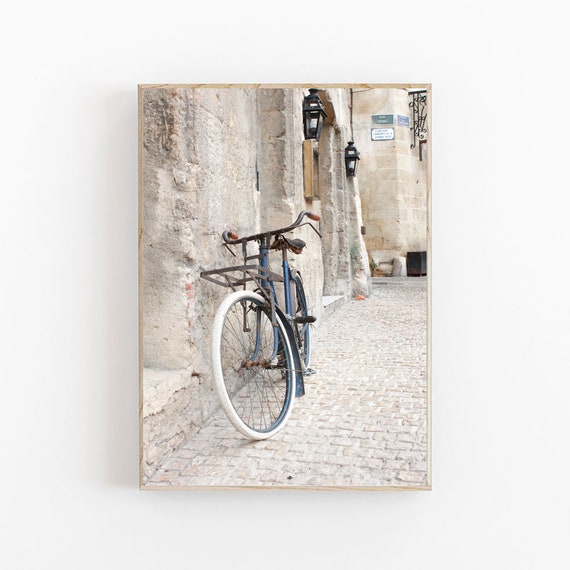The image depicts a beautifully rustic scene of a vintage blue bicycle with brown leather seat and handlebars, leaning against a weathered white brick wall. This wall, characterized by chipped paint and old mortar, lines a curving cobblestone street, capturing the charm of an old European or Mediterranean village. The scene emanates a light, almost white color palette, enhancing its timeless and historic allure. Street lamps adorn an entranceway on the left side, and small, nearly unreadable signs hint at the subtle activity of the quaint locale. The camera's low angle position emphasizes the cobblestone path which appears aged and pale, complementing the unrefined, stony look of the building's façade. The bicycle, with thin wire spokes and a front basket, is central to the composition, its front wheel pointed slightly downward along the alley.